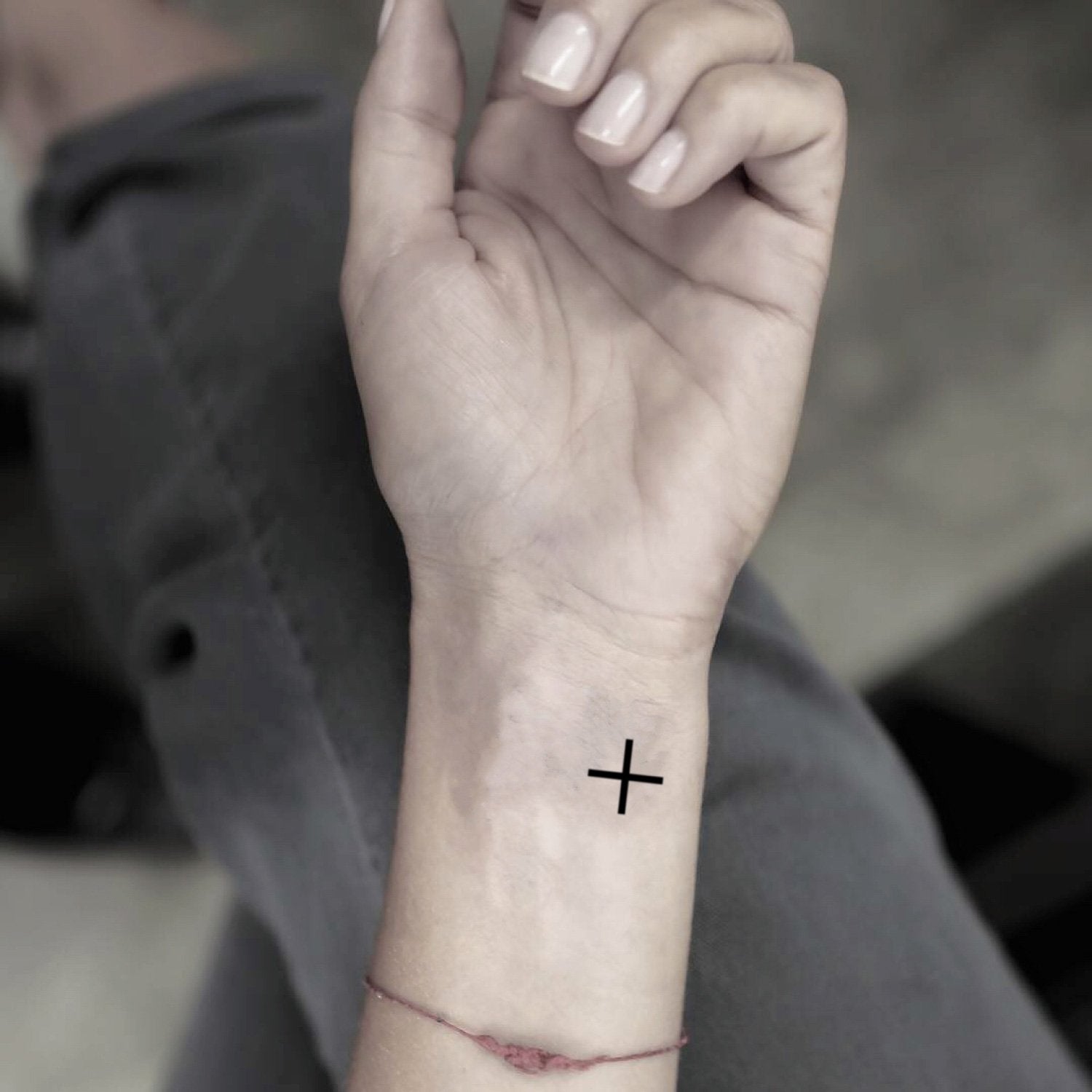The image depicts a left hand, likely of a Caucasian woman, resting atop a crossed leg. The person is wearing dark jeans. The hand has short, well-manicured nails with a glossy, clear or light pink polish. A striking black cross mark is visible beneath the palm. The wrist is adorned with a thin, red rope bracelet. The overall view is from a top-down perspective, capturing the light skin of the arm and the contrasting dark trousers.